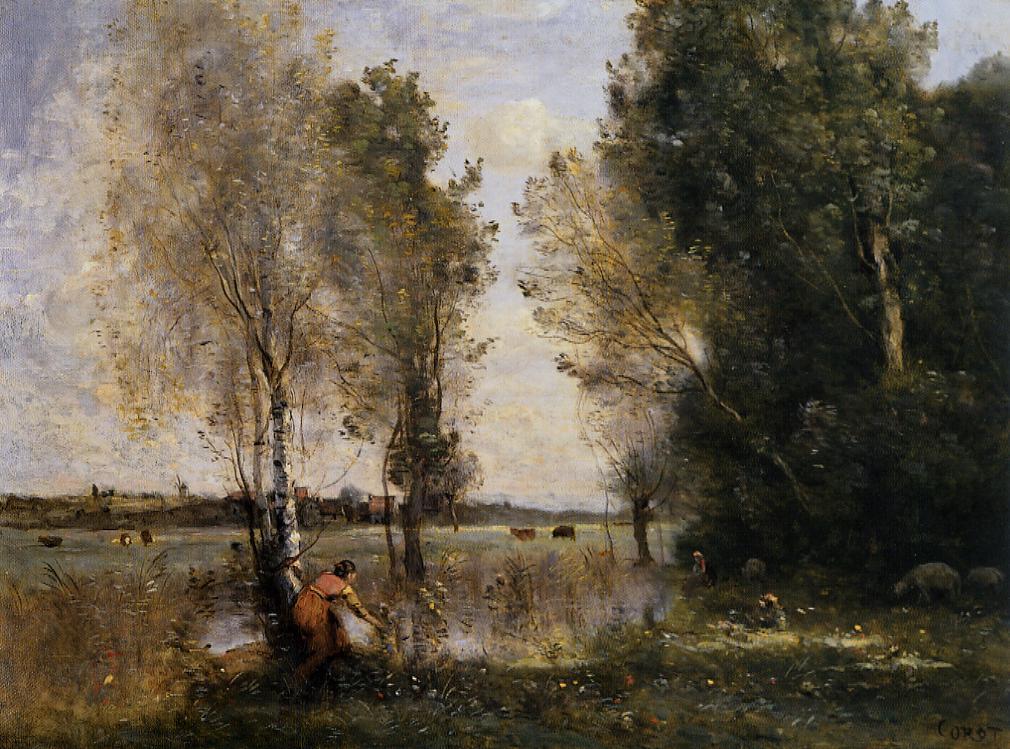The painting depicts a tranquil pastoral scene featuring a woman in a rust-colored dress, standing in a lush field of wildflowers. She is delicately reaching down with her right hand to pick a white flower. The scene is framed by several towering trees, including a white birch tree blooming beside her. To her right, a small group of cows grazes lazily, dispersed in the open pasture that stretches to both sides of the image. In the distance, a serene body of water is shrouded in morning fog, capturing the early hours of the day. Beyond the water, the landscape features a few houses, a hill, and what appears to be a windmill, adding to the idyllic rural setting. The sky above is a mix of blue and lavender hues, dotted with clouds, enhancing the overall sense of calm and peace in the painting.